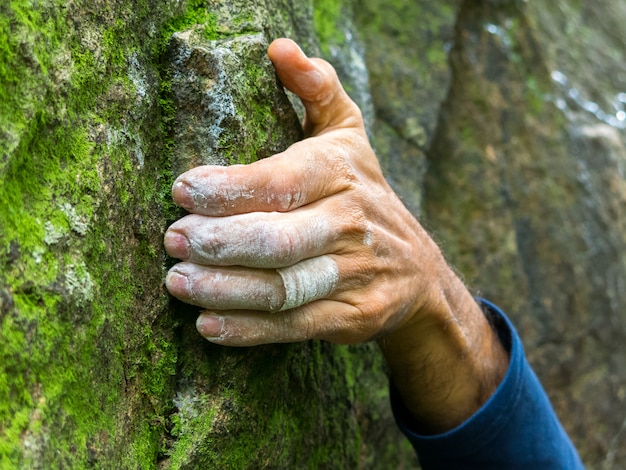This photograph depicts a close-up of a man’s left hand gripping a rough, moss-covered rock face with a background suggesting the side of a mountain. The hand, weathered and strong, features fingers coated in white chalk, with noticeable redness through the chalk, indicating the pressure of the grip. A bandage is wrapped around his ring finger, and his hairy arm extends down to a blue sleeve, suggesting he is engaged in climbing. The rock surface is particularly detailed, with green moss spreading from the lower right to the upper left, enhancing the rugged and lifelike ambience of the scene. The overall impression is one of intense physical effort and connection with the natural environment.